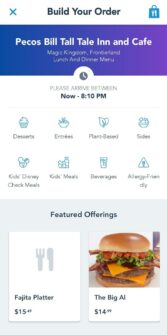The image is a blurry screenshot of a food ordering app interface. At the top center of the screen, the header reads "Build Your Order." Below this header, the text "Echos, Build, TallTale Inn and Cafe" is displayed, indicating the restaurant name. The timeframe "Now, 8-10pm" is also visible beneath the restaurant name, suggesting the current available delivery or pick-up window.

Further down, several categories for food items are listed, including "Beancuits," "Meals," "Beverages," "Allergy Free Sides," "Plant Based," "Entrees," "Desserts," and "Kids." On the left side of the screen, the item "Fajita Platter" is listed, and to the right, "The Big Owl" can be seen, likely referring to another menu item or meal option.